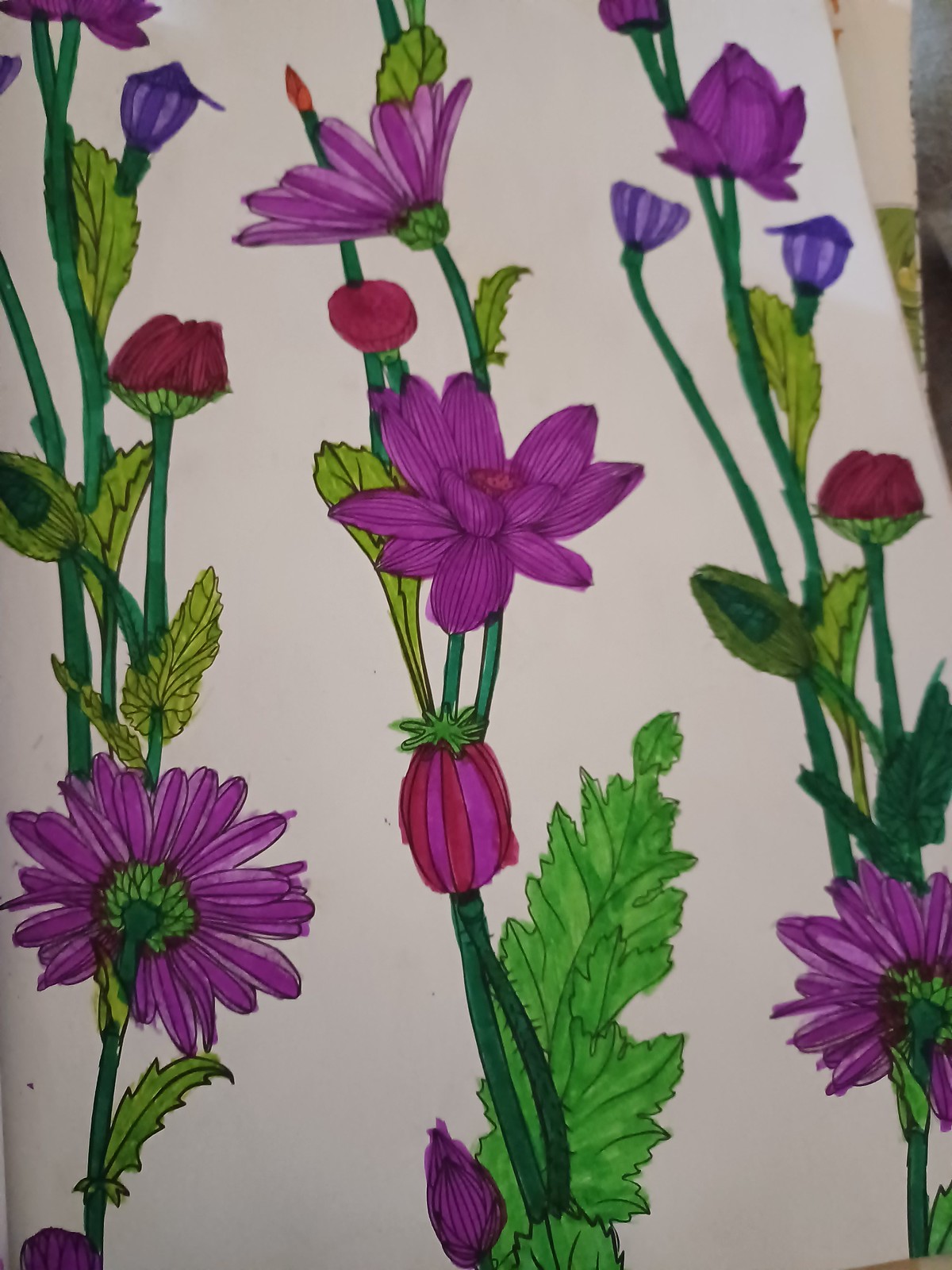This is a detailed drawing of flowers on a white piece of paper, with details partially extending to a secondary paper with green edges visible at the top right, and a white towel-like backdrop behind it. The image prominently features three vertical rows of vine-like stems, each characterized by dark green stems and lighter green leaves. These rows showcase a variety of flowers and buds in different stages of bloom. The flowers are mainly purple with variations including deep pink-purple hues. 

The first row includes a green stem with a purple flower at the bottom facing away, lighter-colored leaves, and another purple flower that hasn't fully opened towards the top. The second row displays a similar dark green stem with a large green leaf and two partially opened purple flowers, one of which has a green top, and a fully open purple flower facing the viewer. The third row features green stems with light green leaves and two darker purple flowers at the top, as well as a bottom purple flower facing away.

Additionally, there are elements of variety with medium-sized red flowers tightly closed, some appearing as fist-tight buds. There are also flower buds in various stages of development, adding to the dynamic nature of the composition. Each stem occasionally emerges with a flower or bud, including some small purple and striped flowers and even a distinctive daisy-like purple flower. The meticulous detailing and varied presentation create a vibrant and intricate floral depiction.